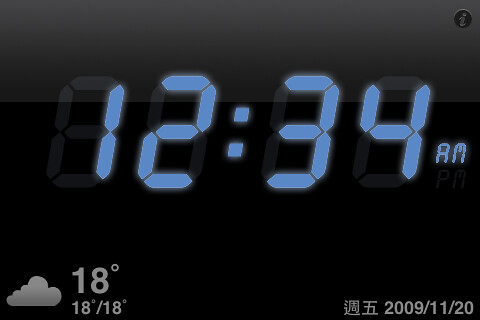The image captures a digital clock display, possibly from a phone screenshot, featuring a traditional alarm clock design with green digital numerals. The time reads 12:34 AM, depicted in the recognizable segmented style of classic alarm clocks. At the bottom left, the display shows a temperature of 18 degrees, indicated by a small cloud icon, suggesting cold and cloudy weather conditions. The date is also present, formatted in the year-month-day style as 2009-11-20, accompanied by a foreign language symbol.